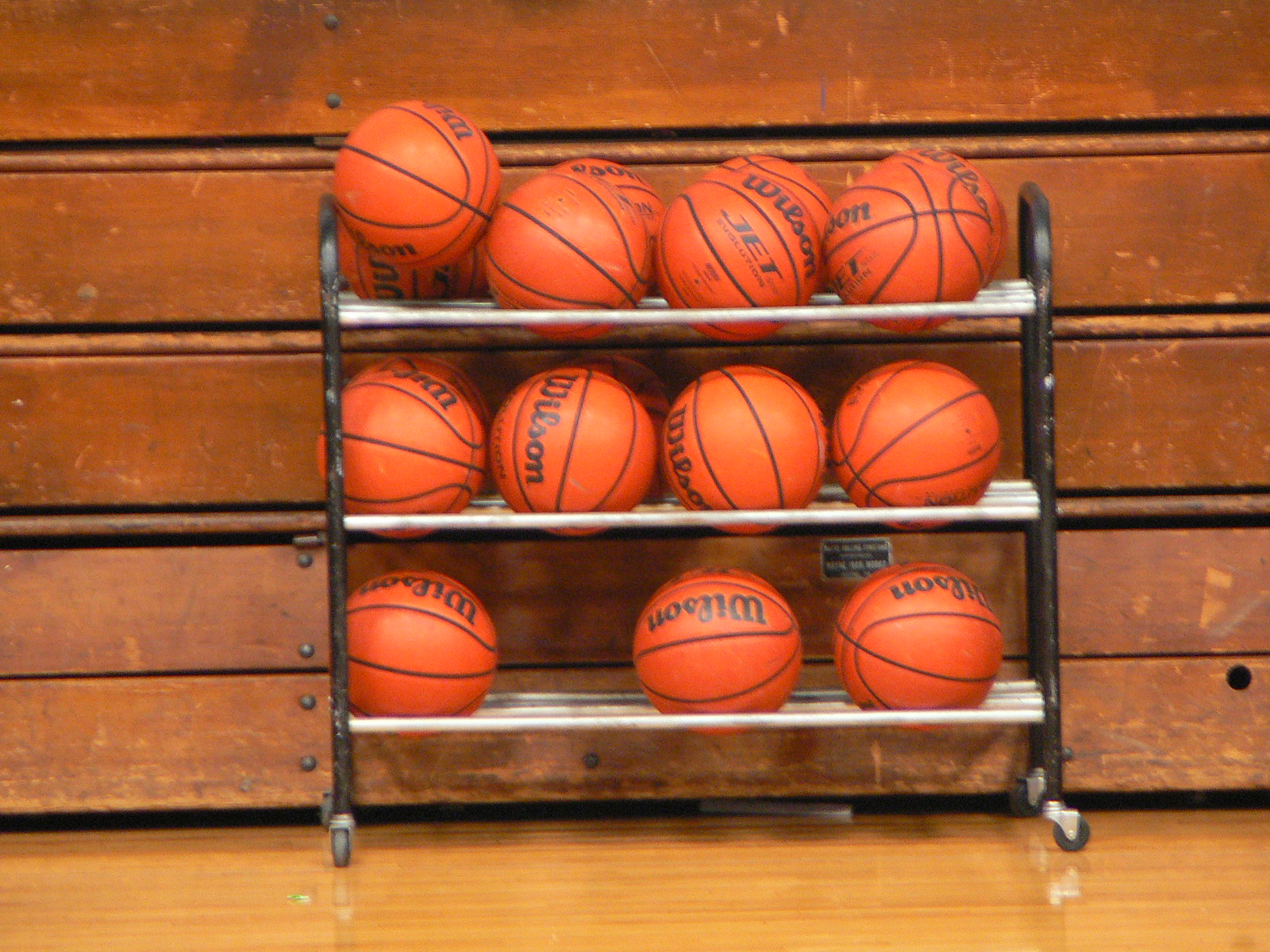In this photograph, a metal basketball rack is prominently displayed, set against folded, wooden bleachers in a gym. The rack, made of chrome with black metal hoops, features three shelves, each structured with two rows. It is equipped with small black wheels, enabling easy mobility. The top and middle shelves each hold four Wilson basketballs, arranged in two rows, while the bottom shelf contains only three basketballs. All the basketballs are standard orange with black piping, branded with "Wilson" and "Jet" in black script. The gym’s high-gloss, light-colored wooden floor reflects the neatly arranged rack, emphasizing the setting’s polished appearance. The worn, brown wooden bleachers, stacked and compressed, add a touch of vintage charm to the otherwise modern facility.